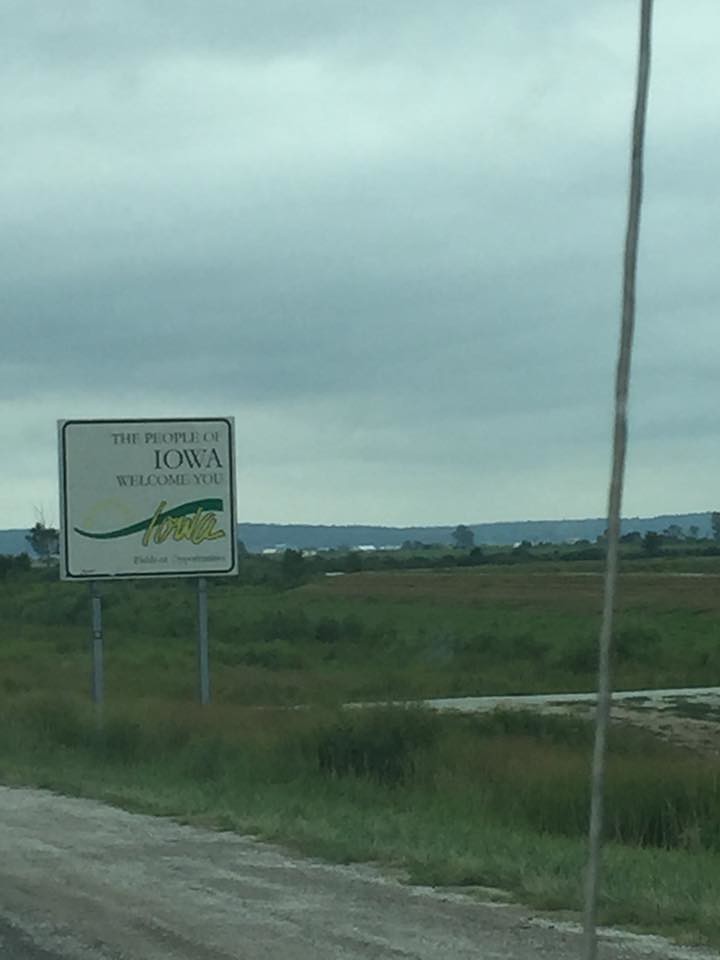Beneath a blurred, gray sky, a sign on the left side of the image prominently displays the words "The People of Iowa Welcome You" in a white square. This sign features a yellow stripe with "Iowa" written on it. The middle and right sections of the image are dominated by lush green, tall grass. In the bottom left corner, a dirt road stretches across the scene. The background showcases a majestic mountainous region, while a solitary stick juts out of the ground to the right. A white pathway intersects with another dirt road, bordered by trees that stretch across the backdrop, completing the serene landscape.